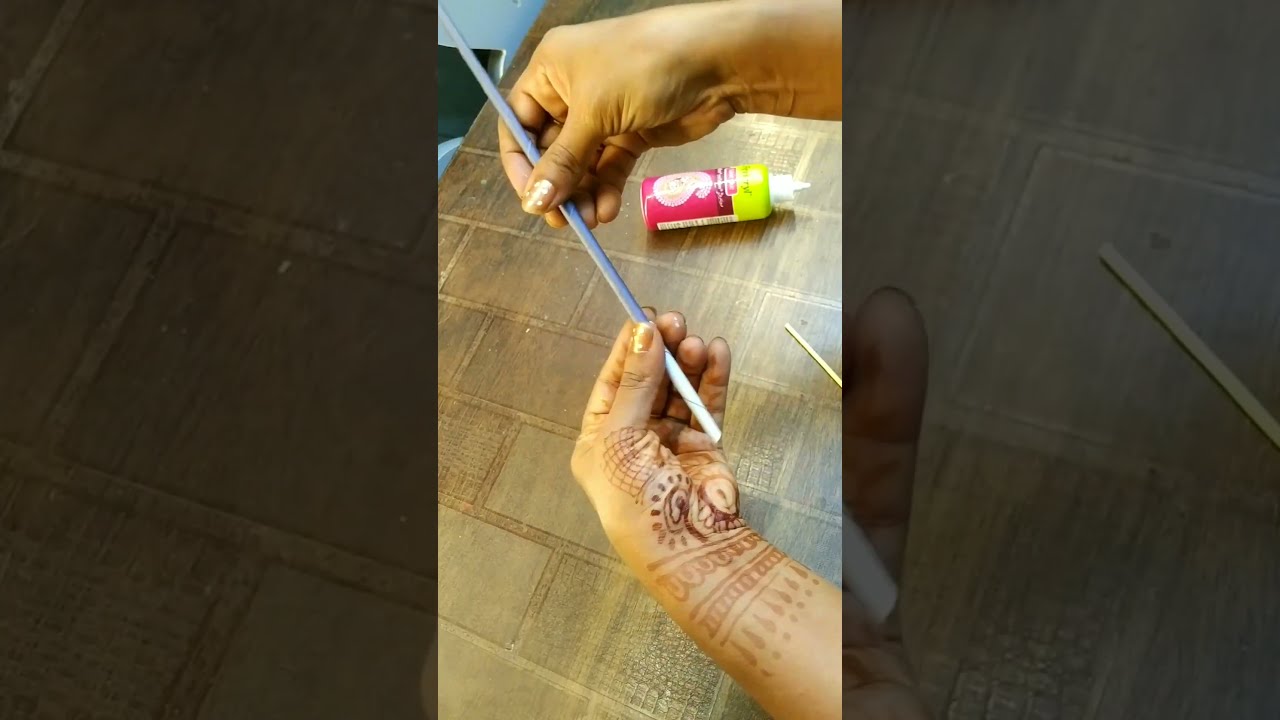The detailed image presents a color photograph in portrait orientation, superimposed onto a darker, landscape background of the same scene. Central to the picture are two hands adorned in intricate henna tattoos extending from the palms to the wrists. The fingernails are painted in a gold color. The upper hand grips a gray rod with a white paper tip, while the lower hand, palm-up, showcases the henna designs. The hands rest on a dark brown table with a brick-pattern laminate that has a greenish tint. A small bottle, possibly of glue, lies on its side beneath the hands. The bottle features a light green and pink label with a white flip cap. Wide dark borders frame the central image on either side, adding to the overall composition's photographic realism.